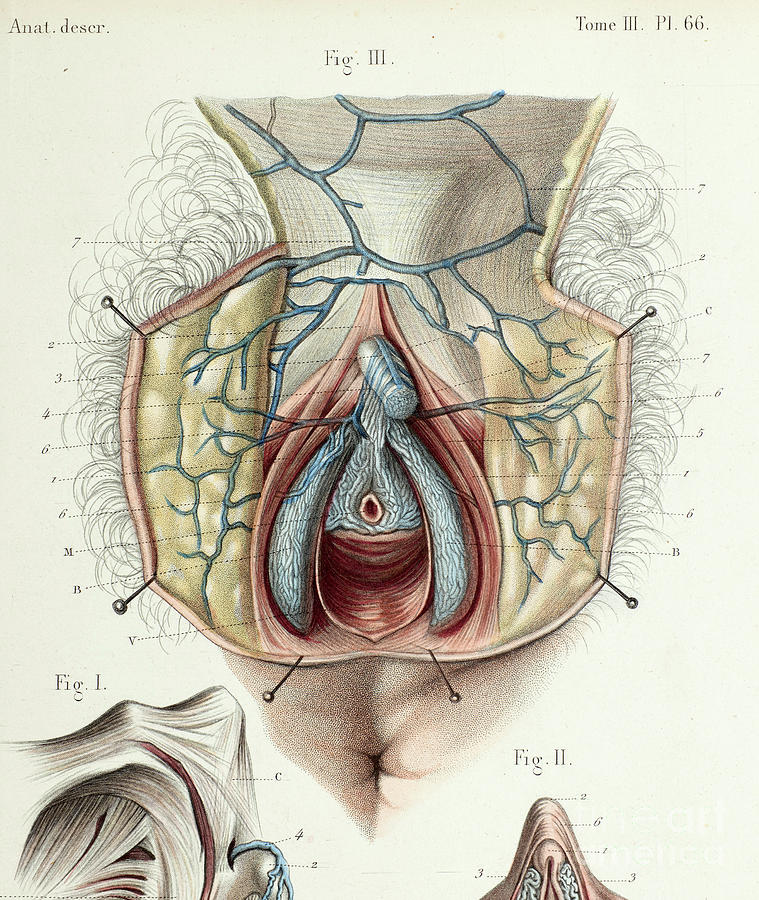This is a detailed, colored anatomical illustration from the late 1800s to early 1900s, depicting the dissected female anatomy. The background is an ivory color. In the top left corner, it is labeled "anat.descr.", likely short for "anatomy description." The illustration is divided into sections labeled "figure 1," "figure 2," and "figure 3." 

"Figure 1" shows tendons and blood vessels with blue veins, detailed near the birth canal. "Figure 2," located at the bottom right corner, offers a close-up of additional anatomical structures, featuring more veins and labeled points. "Figure 3" seems to represent a leg, with anatomical markings leading to it. 

The diagram reveals internal areas with the skin pinned open, displaying the birth canal and rectum area, along with a decipherable drawing of body hair and orifices. The top center of the diagram is marked "tome 3 pi.66.", signifying the specific tome and plate number of the instructional material. The overall intent of the image is to provide a detailed educational view of the internal female anatomy, including the vaginal and rectal regions, highlighted with meticulous numbered labels for instructional purposes.